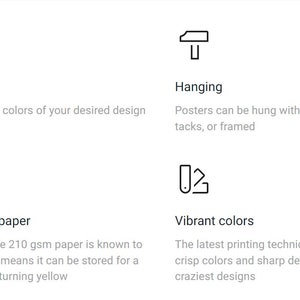This digital screen displays an informational graphic divided into four distinct sections, arranged in a two-by-two grid. The background is predominantly white, providing a crisp and clean canvas for the detailed content. 

In the top left section, written in gray, is the header "Colors of Your Desired Design," presumably introducing the color palette options for a given service or product. 

Adjacent to this, in the top right section, there is an icon resembling a peg, accompanied by the word "Hanging" in bold black text. Below it, in smaller gray text, are instructions: "Posters can be hung with tacks or framed."

In the bottom left section, the large black text reads "Paper," and beneath it, though partially obscured, the gray text seems to reference the durability of 210 GSM paper, likely indicating that "it can be stored for preventing yellowing," although the exact text is cut off.

Finally, the lower right section features a visual of rectangles fanned out, symbolizing a variety of options. The bold text here states "Vibrant Colors" and is followed by gray text that highlights the use of "the latest printing technique" for "crisp colors and sharp details," emphasized by the phrase "Craziest Designs."

Overall, the image effectively communicates aspects of design, hanging options, paper quality, and printing techniques with a structured and visually appealing layout.